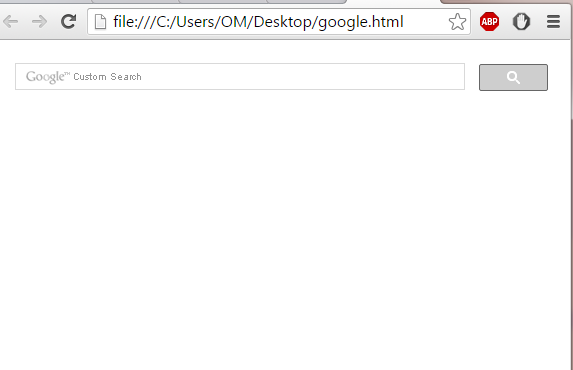A detailed screenshot displays the upper right corner of a web browser interface. The main section of the browser is empty, devoid of any content or search results. The focal point is a Google search box situated prominently within the browser's blank body. The search box features the recognizable Google logo accompanied by the text "Custom Search," and is flanked to the right by a gray search button.

In the upper right corner of the browser, the familiar three-bar menu button is visible, signaling access to additional browser options. To its immediate left is a grayed-out button displaying a hand icon, likely indicating an active browser extension, possibly NoScript. Adjacent to this is the Adblock Plus icon, signifying that the ad-blocking extension is installed and functioning.

To the far left is the browser’s address bar, currently showcasing the text "file:///C:/Users/om/Desktop/google.html." This reveals that the user is accessing a locally stored HTML file, which hosts a custom Google search engine. Below the address bar is the Google search box, reiterating the "Custom Search" functionality. The overall image highlights a personalized setup, showcasing extensions like Adblock Plus and NoScript, within a custom local HTML environment for Google searches.